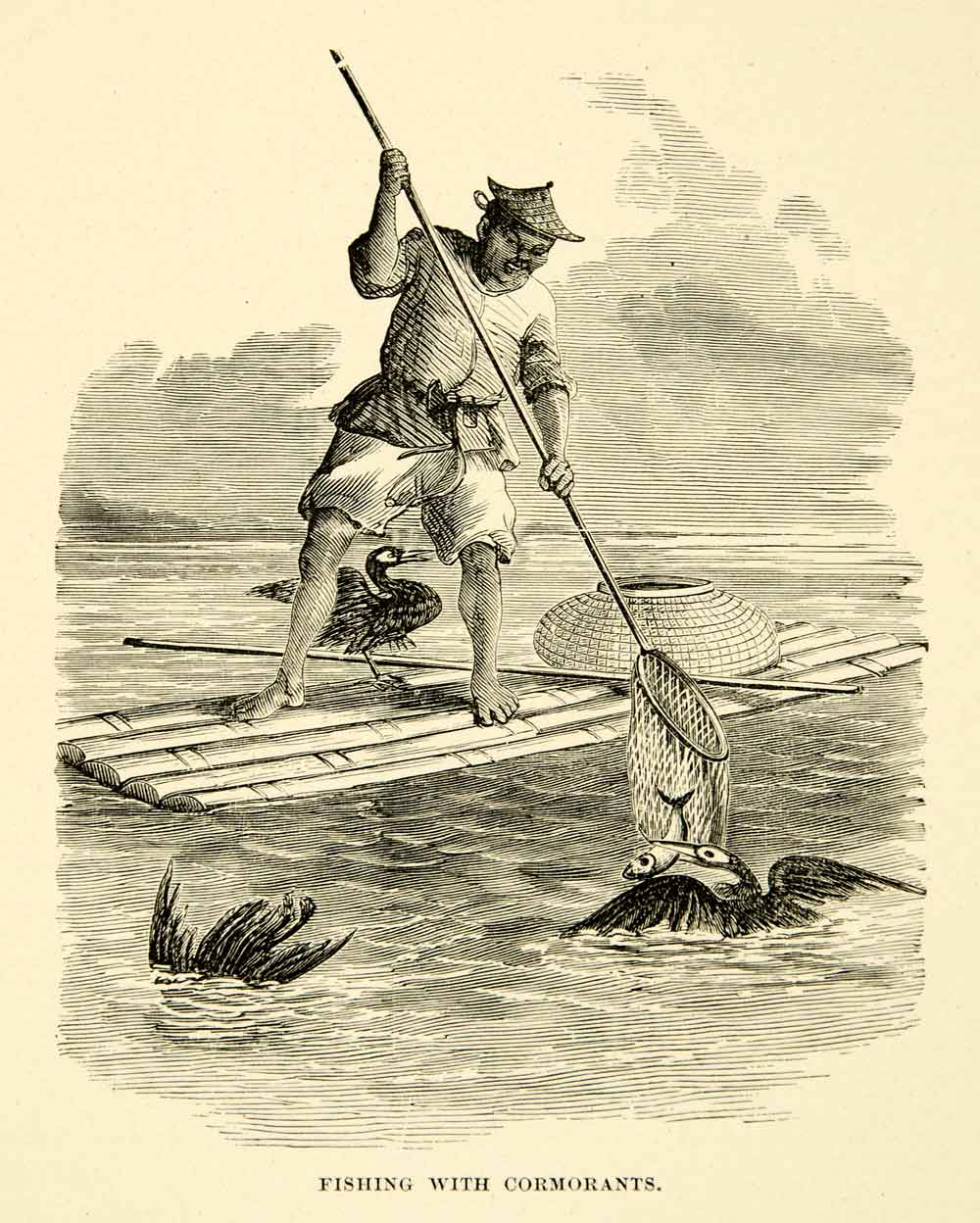The image is a black and white, hand-drawn illustration resembling a vintage postcard or an old book illustration. It depicts an Asian fisherman, likely Chinese, standing on a narrow bamboo or wooden raft. He is dressed in traditional clothing, with shorts that go above his knees, and wears a distinctive, conical bamboo hat. The fisherman is barefoot and holds a long pole with a net at the end, which he appears to be using to catch fish. 

In the water near the net, a cormorant bird has caught a fish in its mouth, while another cormorant dives beneath the surface. A third bird is perched on the raft behind the man. The scene is set against a backdrop of wavy water patterns and a cloudy sky, drawn with line techniques. There's a wicker basket on the raft, intended for storing the catch, although the birds seem to be thwarting his efforts, as suggested by the text at the bottom of the image: “Fishing with Cormorants.” The entire composition is rendered in meticulous black and white ink, giving it a timeless, monochromatic aesthetic.